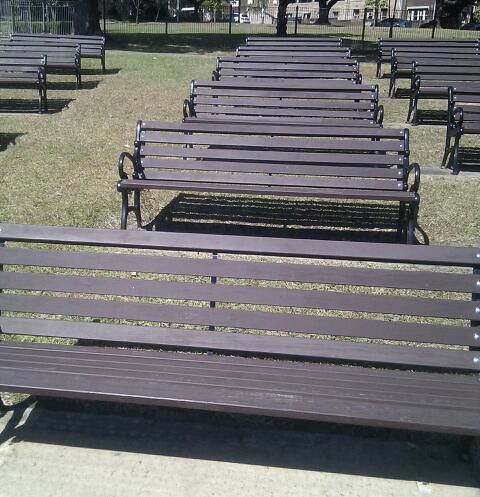The image captures an expansive, well-manicured lawn in a park-like setting, bathed in sunlight. Central to the photograph are rows of dark brown wooden benches with black metal legs and armrests, precisely arranged in a formation reminiscent of an outdoor amphitheater or seating for an event like a play or a wedding. The primary row, consisting of six benches, stretches prominently from the foreground deep into the image, flanked on the left by a set of three benches and on the right by four benches. Each bench, capable of seating four people, is constructed with horizontal wooden slats separated by black metal framework. Ample grassy aisles provide pathways between the rows. Behind this orderly assembly, a tall black fence stands sentinel, with a few trees peeking over it, and in the far background, large buildings loom, adding a sense of scale and context to the serene, open space.